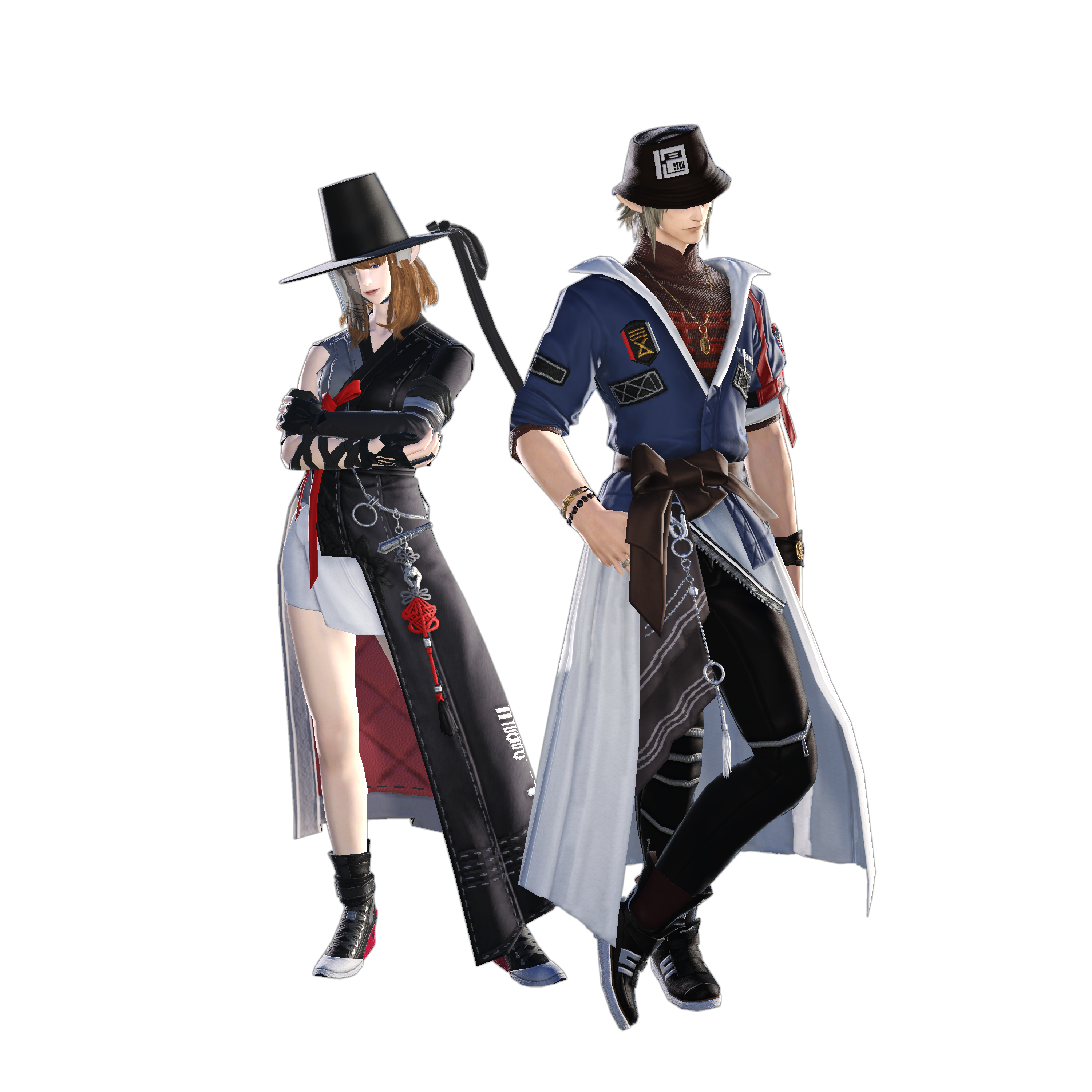The image depicts two in-game characters styled in a Japanese animated, vaguely steampunk aesthetic, standing against a blank white background. On the left is a woman with pale white skin, adorned in a tall black top hat with a wide brim, featuring a black rope hanging from the left side. Her hair is long and blonde, cascading from the top of her head. She wears a long, black leather jacket that drapes to her ankles, open on her left side and exposing her right arm. The jacket is detailed with a red string arranged in the shape of a rose. Her attire includes a short white skirt, black Converse-style sneakers with white soles and red heels, and black socks. 

To her right stands a slightly taller male character with white skin and silver hair, which is short and shaggy. He sports a black top hat similar to the woman's. His outfit consists of a blue sweatshirt jacket rolled up to the elbows and unzipped halfway, a gold necklace around his neck, a white blouse tied around his waist as a cape, and a broad brown belt. He completes his look with black pants and sneakers akin to those worn by the female character. Both characters have long, elongated pointy ears reminiscent of elves.